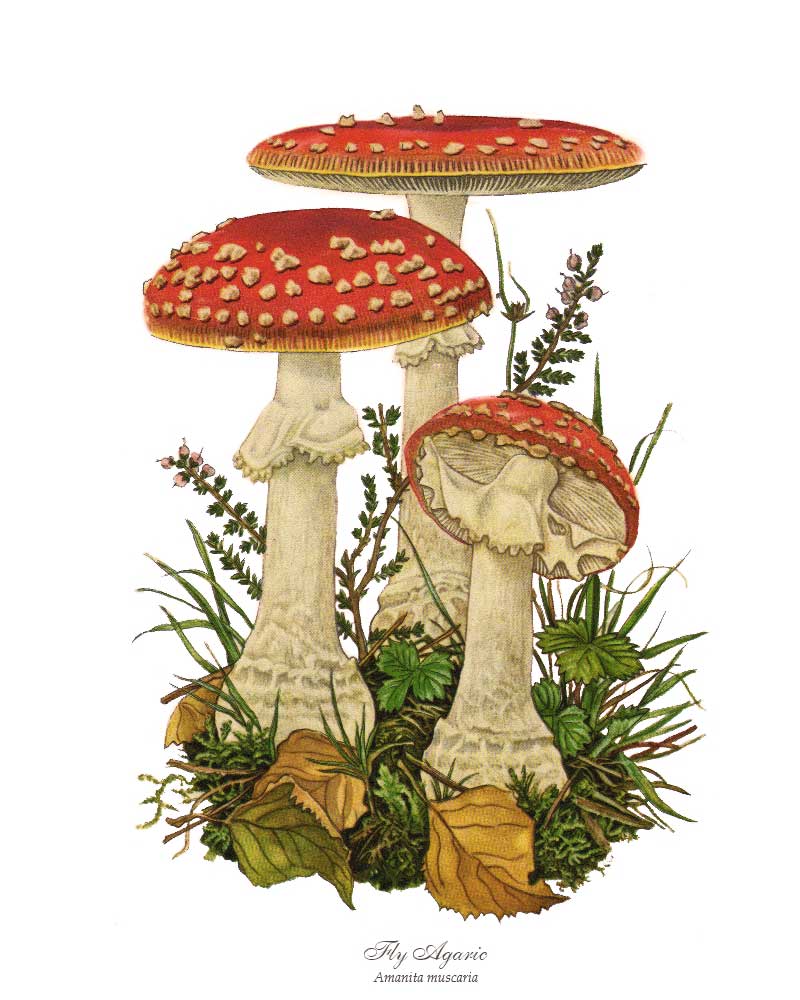This vibrant and beautifully detailed illustration depicts a group of three Fly Agaric mushrooms, scientifically known as Amanita muscaria, as indicated by the script at the bottom of the image. The mushrooms are characterized by their striking red caps adorned with white specks, each varying slightly in height and shape. The tallest mushroom stands at the back with a broad, round cap, the middle one is slightly shorter and almost as broad, and the smallest one tilts slightly, exposing its gill structure beneath the cap. The mushrooms are set against a lush background of green foliage and grass, interspersed with brown and dead leaves, as well as some thistle. The scene is richly colored, with the mushroom caps featuring accents of gold around the edges, enhancing the overall aesthetic of this traditional illustration.